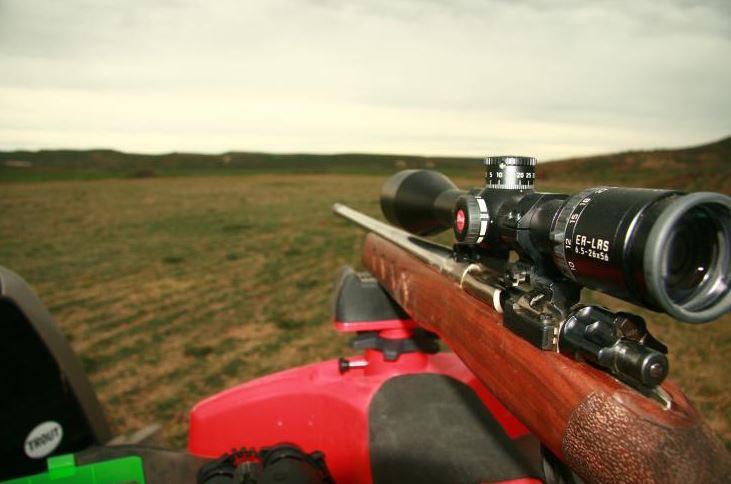The image depicts an outdoor scene featuring a hunting rifle prominently displayed on a red and black vehicle mount. The rifle itself has a wooden stock and a long silver barrel, complemented by a black scope on top. This scope features a circular ring with white numbers, including 5, 10, 12, 15, 18, 20, and 25, and is marked with ER-LAS 6.5 to 25 by 56. The rifle is resting on a brown wooden surface, possibly a pole, which is integrated into the vehicle mount. In the foreground, there is a field with a mix of green and yellowish-brown grass, while the background showcases a range of hills or mountains. The sky above is mostly gray with many clouds, giving the entire scene a slightly overcast appearance. In the bottom left corner, the word "trout" is visible in black on a white circle, accompanied by a green clip-like object.